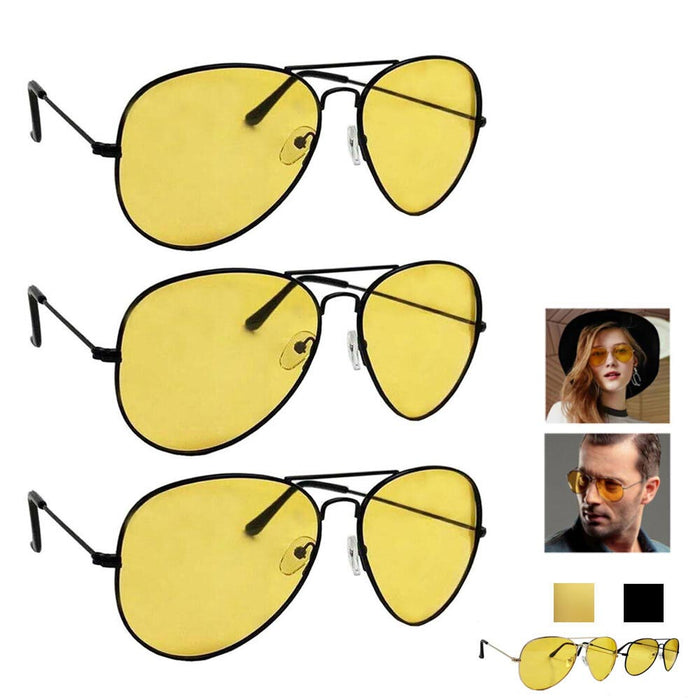The image is a square-format product photograph showcasing aviator-style sunglasses. Central to the image are three repetitions of the same pair of wire-framed sunglasses, stacked vertically against a white background and facing diagonally to the right. The frames of the sunglasses are composed of thin black wire, and the lenses are a light green or yellowish tint, designed to be transparent. Each pair features a visible nose piece and ear pieces that curve downwards.

On the right-hand side of the image, there are two smaller photographs of models. The top photo features a stylish woman with long blonde hair, parted to the side, wearing a black wide-rimmed hat and looking slightly downward. She is also wearing a pair of the featured sunglasses. Below her is a photograph of a man with short dark hair, slicked back, and closely trimmed stubble on his face. He, too, wears the same sunglasses, giving off a sophisticated look.

Underneath the models' pictures, there are two color swatches: one pale green, matching the lens color, and one black. Below these swatches, two more pairs of sunglasses are displayed, one with a gold wire frame under the green swatch, and one with a black wire frame under the black swatch, enhancing the visual representation of available frame colors. The overall style of the photograph is realism and product representationalism, showcasing the detailed design and color variations of the sunglasses.